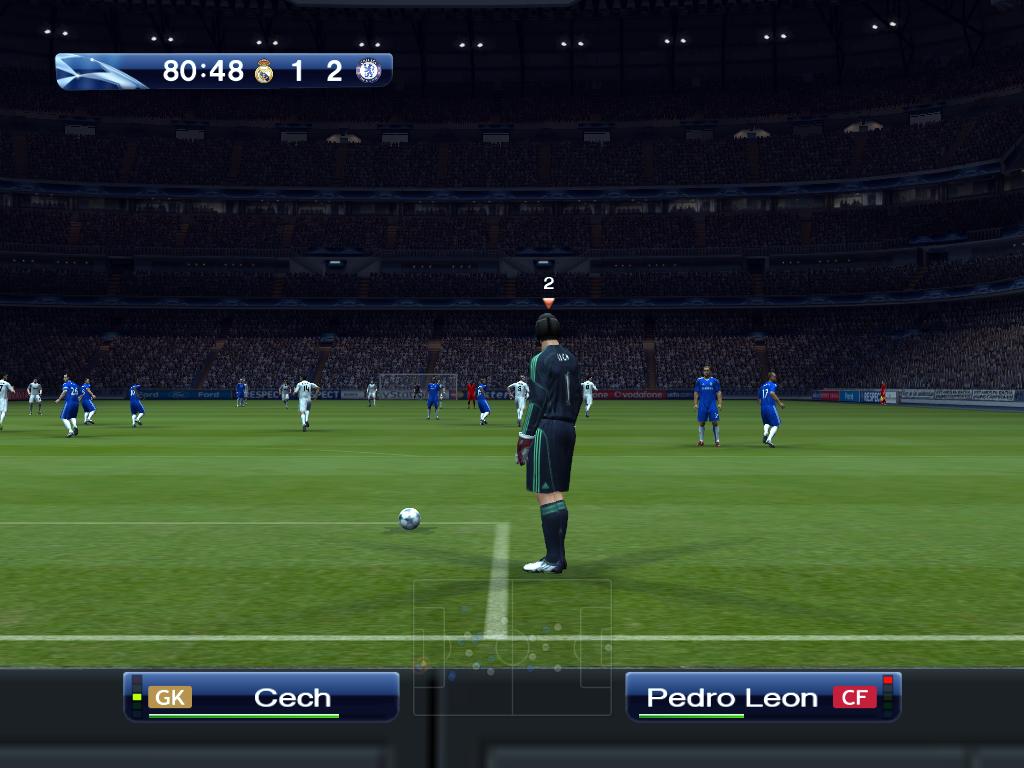The image depicts a highly realistic FIFA soccer video game. At eye level, we see a vibrant green field with crisp white chalk marks. Standing center stage is a player poised to kick a ball positioned just to the right of a chalk outline box. This player, marked by the number 2 above his head, wears a black shirt with green accents, matching black shorts, tall black socks with green tops, and white cleats. His left hand sports a sizable glove. The player gazes at his teammates in the background. The field is bustling with players in either blue or white uniforms. Behind them, a four-level stadium packed with animated crowds is visible under the shadowed upper stands dotted with tiny lights.

In the lower left corner of the screen, text reads "CECH" next to a green health bar and an orange "GK" label. On the right, it says "PEDRO LEON" with a partially filled health bar and a red "CF" label. A transparent mini-map displays player positions on the field between these text boxes. Additionally, the upper left corner features a blue bar with white text displaying match details "80:48," flanked by circular logos and additional numerical information.